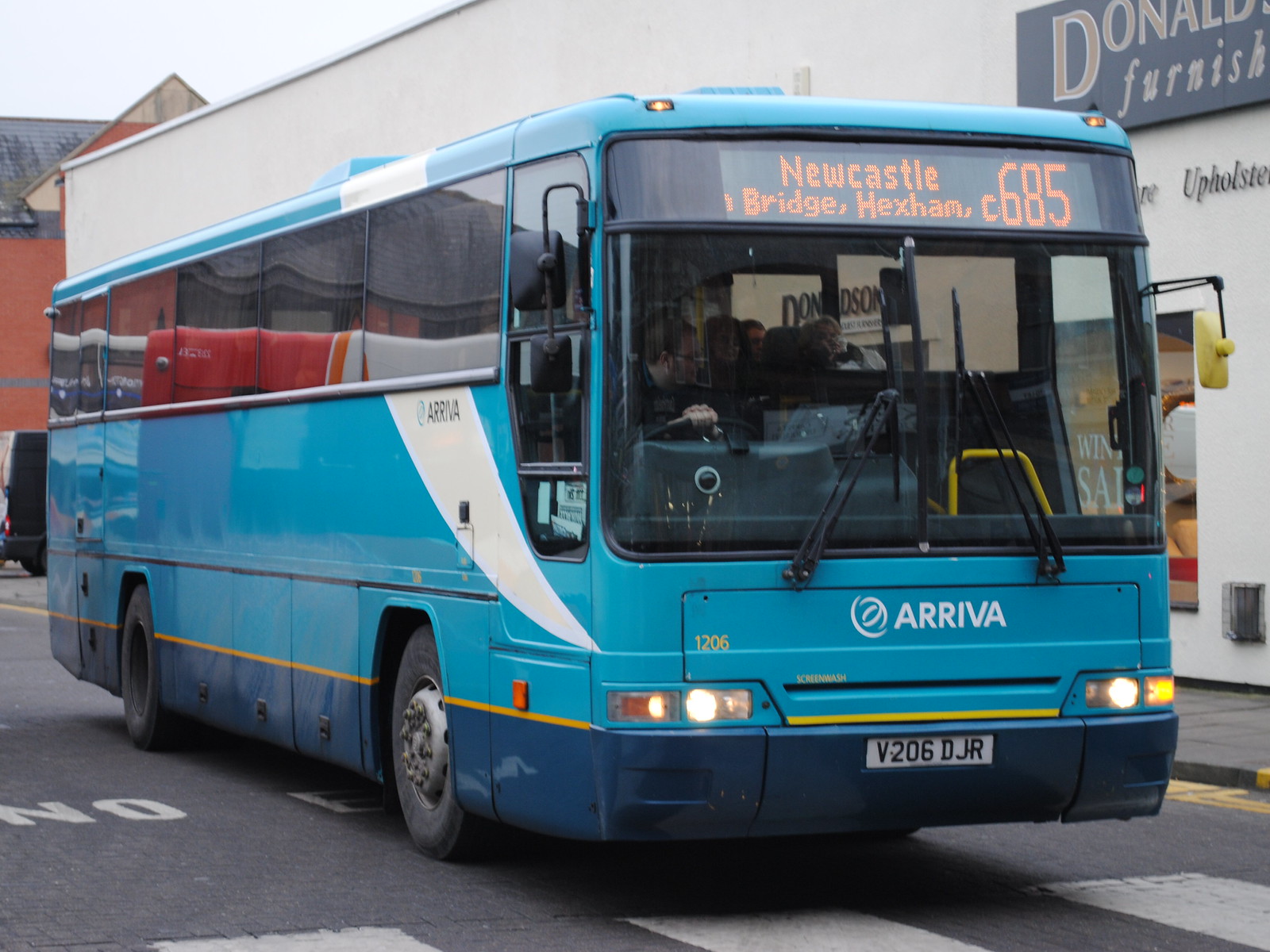In this image, a light blue bus with dark blue accents and a gold stripe along the bottom is prominently featured. The bus has "Arriva" printed in white lettering beneath the windshield, along with a gold number "1206" and "Screen Wash" to the left. Below this, the white license plate reads "V206 TJR." The driver's seat is visible through the large windshield, and the driver has his hand resting on the upper part of the steering wheel. Seated passengers are also visible inside. The information screen above the windshield displays the route "Newcastle Bridge, Hexham, 685."

The bus is either parked or stopped at a crosswalk in front of a store with a sign reading "Donald's Furnishings." This store features white walls and a gray sign at the top. Behind the store, a brick building with a triangular roof is visible, set against a white sky. In the reflection on the bus's windows, a red and white-orange bus can be seen, and a black vehicle is positioned behind the bus.